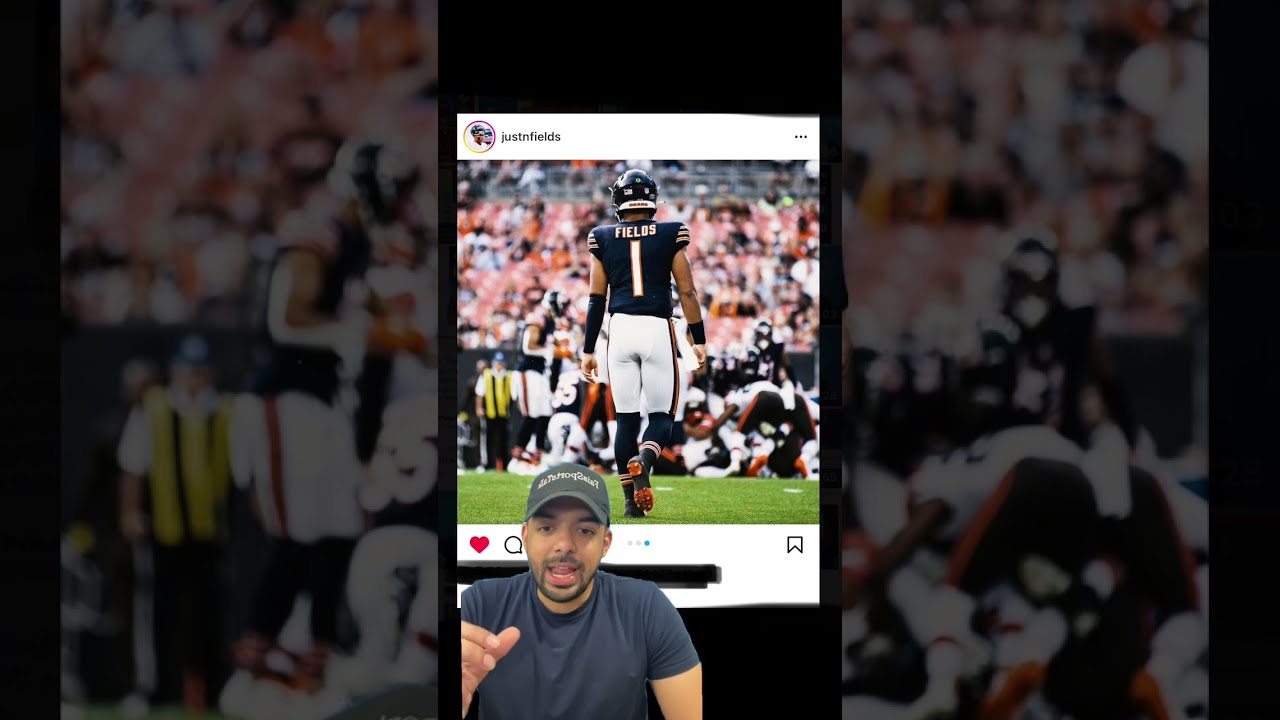The image is a horizontally rectangular composition divided into three vertical sections. The central section features a screenshot from an Instagram post, prominently displaying a football player walking on a field. This player, identified as Justin Fields, is shown from the back wearing a black jersey with white pants and a helmet, while the name "Fields" and the number "1" are visible on his uniform. Surrounding him is a blurred background filled with other players and spectators in the stands.

In the foreground of the central section, there's a man speaking directly to the viewer, seemingly narrating or providing commentary on the football scene behind him. This man, wearing a gray cap and a gray t-shirt, appears to be discussing or reflecting on the action depicted in the Instagram post. His thin black mustache and beard are also noticeable.

The first and third sections of the image consist of darkened, blurry close-ups of the background elements from the central football scene, providing a sense of depth and focus on the main subjects of the Instagram post and the narrating man.